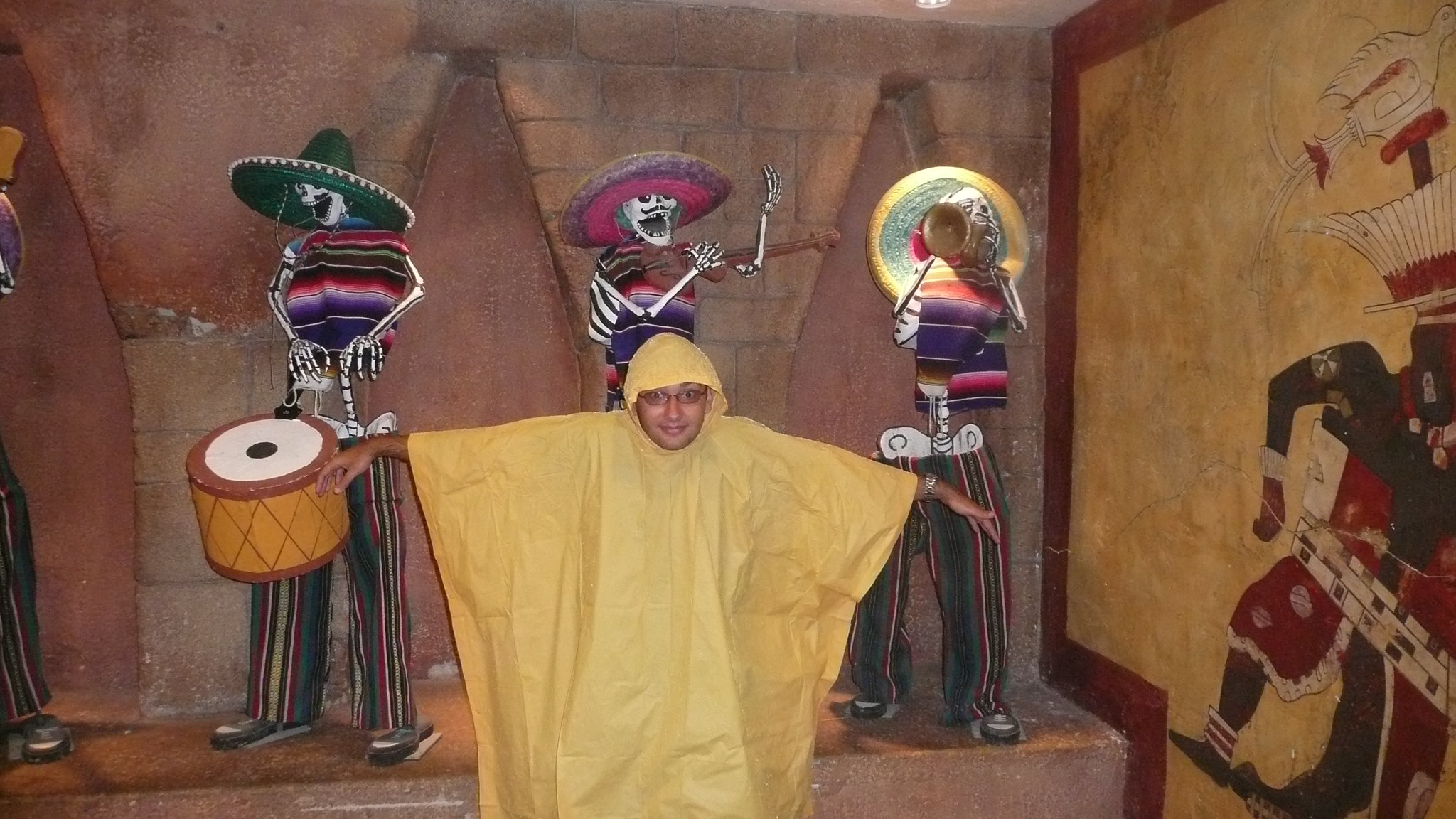This photograph captures a young person, possibly Hispanic, standing in what appears to be a cave-like structure or an underground setting that might be part of a museum exhibit. The individual is wearing a hooded yellow poncho, resembling a raincoat, with their arms extended outward as if ready to embrace. They are smiling toward the camera and wearing glasses. Behind the person, there are three skeleton figures arranged on a brownish brick or concrete slab, dressed in colorful Mexican attire reminiscent of a mariachi band. The skeleton on the left wears a purple, red, and white striped poncho, vertically striped pants in colors of yellow, red, black, and blue, a green sombrero, and holds a yellow and brown drum. The middle skeleton, with a pink and purple sombrero, has its hands raised as if singing. The skeleton on the right, with a yellow sombrero, has its head tilted back, appearing to drink from a gold jug. The background features brown stone walls and, on the right side, a yellow painted wall with a red border and a depiction of a historical figure, possibly from Aztec or another significant cultural era. The overall scene suggests themes related to the Day of the Dead celebration.